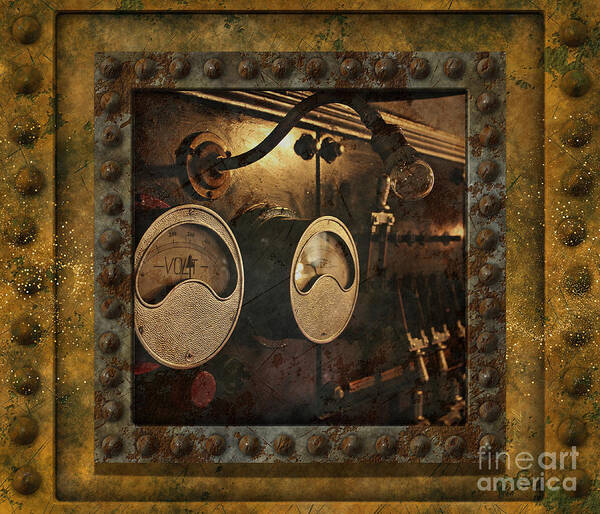The image captures a detailed scene resembling a rustic, steampunk-inspired painting or photograph, possibly framed within a metallic, rusted border reminiscent of an old underwater submarine or sunken ship. The frame transitions from a rusty yellow to a rusty gray hue, adorned artistically with what appear to be screw-like decorations. Central to the artwork is an aged, old-fashioned voltmeter with a straight up-and-down arrow indicator, accompanied by another, less readable circular meter. These meters are set against a backdrop of switches and levers, all contributing to the worn-down, industrial aesthetic. Above the meters hangs a small light bulb on a wire, positioned to illuminate the gauges. A watermark reading "fine art america" in lowercase letters is discreetly placed in the bottom right corner of the image.